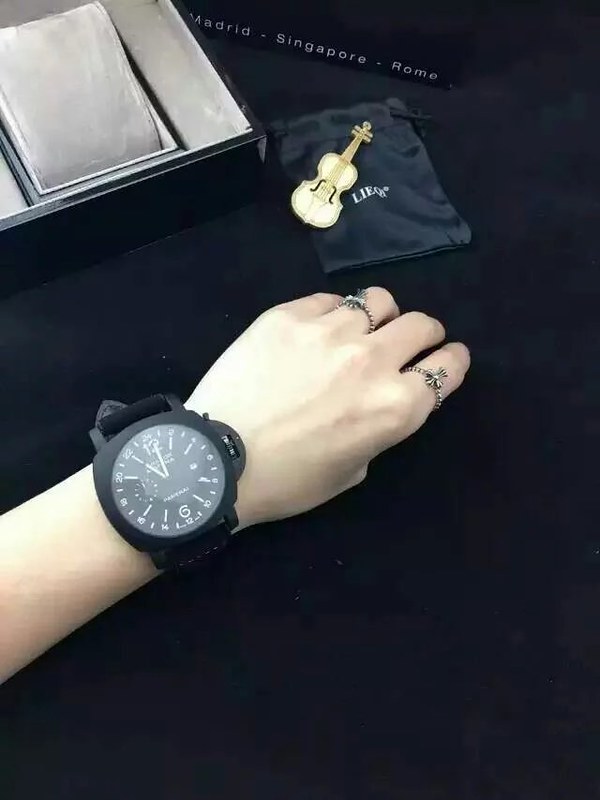A close-up image captures a fairly large wristwatch adorning the left wrist of a man. The watch features a substantial black frame and a matching black wristband. Its face is black, accented with gold lines that mark the hours, but only the numbers '12' and '6' are distinctly present. The man also wears two rings: one on his ring finger and another on his index finger. Above his hand, a small satin bag, presumably for the watch, is visible. The intricate detailing of both the watch and the jewelry adds a layer of sophistication to the overall composition.